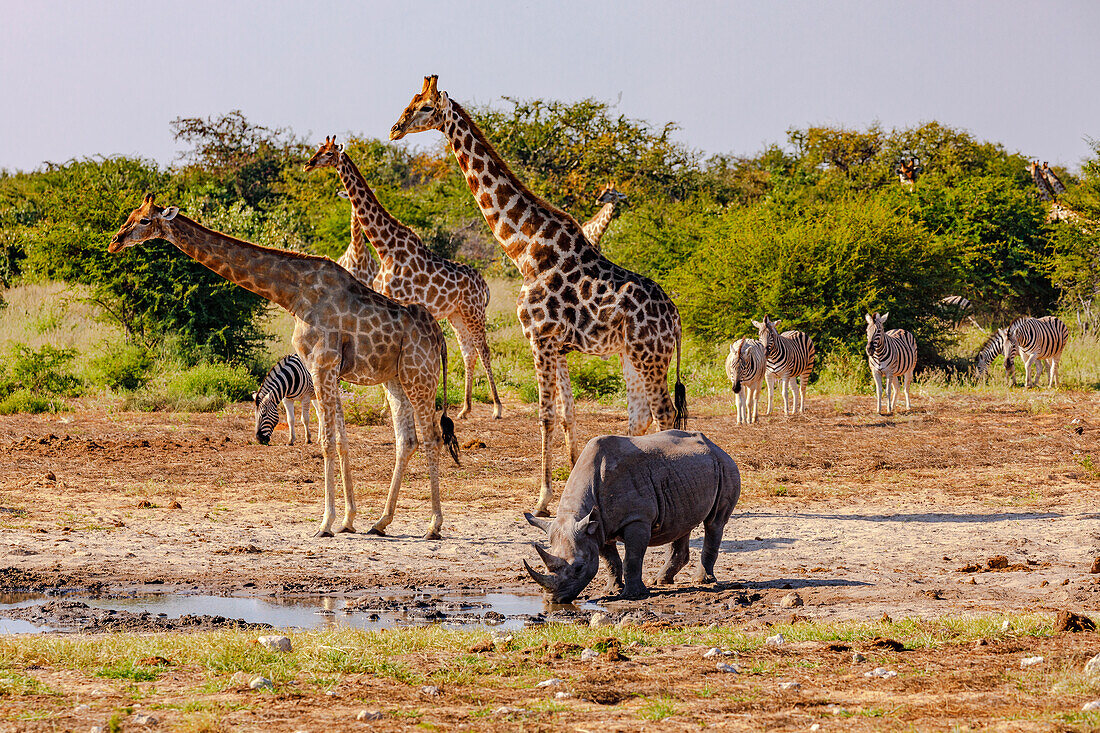In this striking picture taken in a wild area of Africa, a diverse assembly of animals is captured in their natural habitat, possibly within a nature preserve. The foreground features a rhinoceros with two horns, the longer one in front, drinking from a large puddle of muddy water on a stretch of light-brown dirt interspersed with small patches of grass and stones. To the left of the rhinoceros, five giraffes, two males and two females, stand closely together, all intently gazing at the camera. Additionally, there are more giraffes spotted in the background, some nibbling on the leaves of the tall, dry-looking trees that form a backdrop for the scene. Behind the giraffes, a pack of six zebras, distinct with their black and white stripes, appears; one zebra is seen grazing while the others are motionless, also looking at the camera. The sky above is a pale, almost silvery-blue, casting a serene light over the gathering of these magnificent creatures.